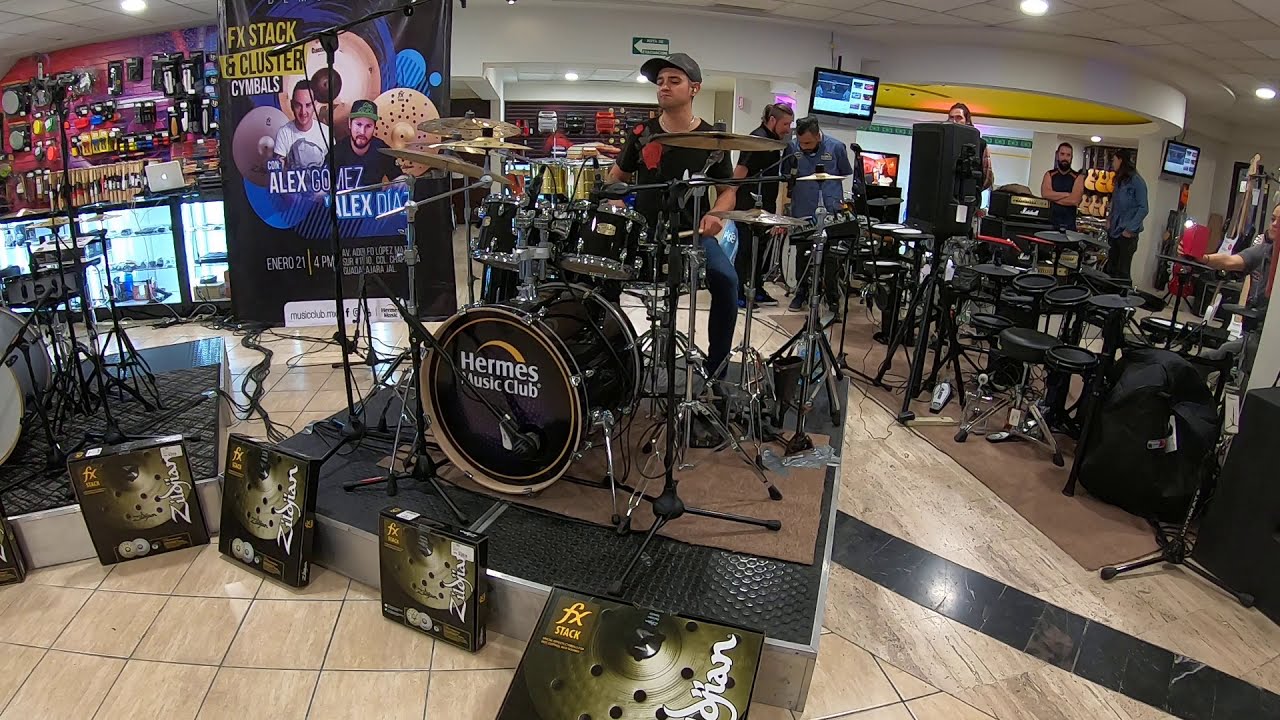The image showcases an indoor setting of a music store or recording studio, where a vibrant scene unfolds in a spacious, rectangular layout. At the center is a square-shaped platform, slightly tilted diagonally, upon which a man sits behind an elaborate drum set. The bass drum, colored black, prominently features the inscription "Air Maze Music Club" (or possibly "Hermes Music Club" due to conflicting text reports). The drum set is surrounded by a variety of cymbals.

In the foreground, several square boxes adorned with the Zildjian brand are stacked, indicating they contain cymbals for sale. The platform is situated on a glossy, beige-tiled floor, and to the left, another platform holds a microphone and various equipment. A comprehensive array of musical instruments spans the store, including flat drums, guitars mounted on the far wall, and percussion instruments. There is also a prominent banner featuring FX stack and cluster symbols, suggesting a product demonstration is underway.

Behind the performer, an array of other musical instruments and accessories, such as drumsticks and maintenance tools, is displayed for sale. A crowd of onlookers, including individuals quietly conversing or focused on the drummer's performance, enhances the atmosphere of a live presentation. Additional elements like a TV screen and posters enrich the background, along with another drum set and a storefront area where a person with a laptop is stationed, indicating a commercial and interactive environment. Overall, the image captures a bustling, well-equipped music store during a live demonstration or event.